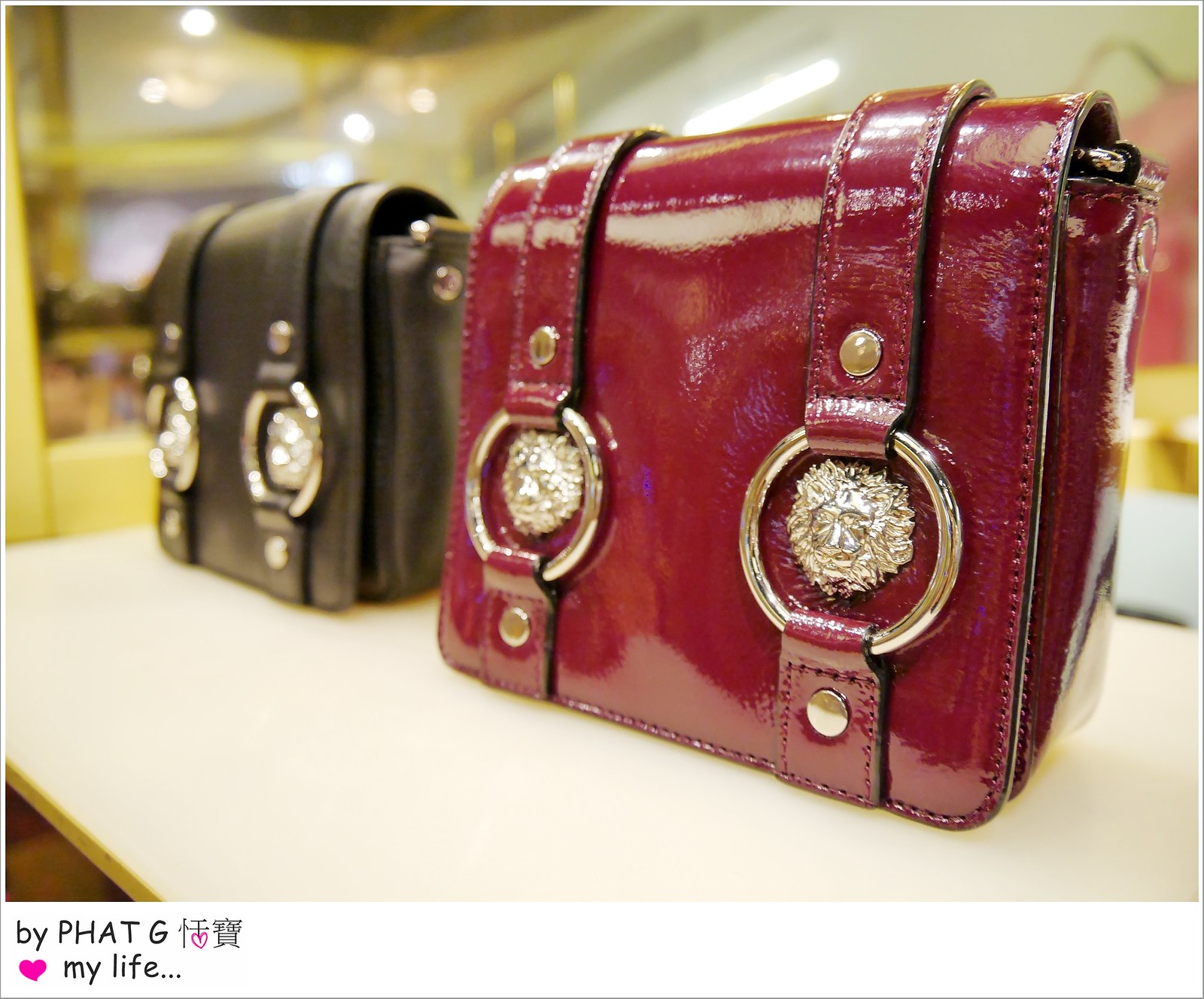The image depicts the interior of a department store, with a close-up focus on a glossy red leather handbag prominently displayed on a white table. The handbag features purplish leather straps, secured by a silver ring at their center. Beneath this ring is a decorative silver lion's head with a large mane. The handbag’s flap partially covers its right side, revealing its glossy purple finish. In the background, slightly out of focus, there is another similar handbag in black. The top portion of the image shows a hint of the store environment, including glass enclosures, stands, and a faint outline of a mannequin or hanger with what might be a red or pink shirt. At the bottom left corner, the text "by PHATG" is visible, followed by Japanese symbols, a pink heart, and the phrase "my life..."